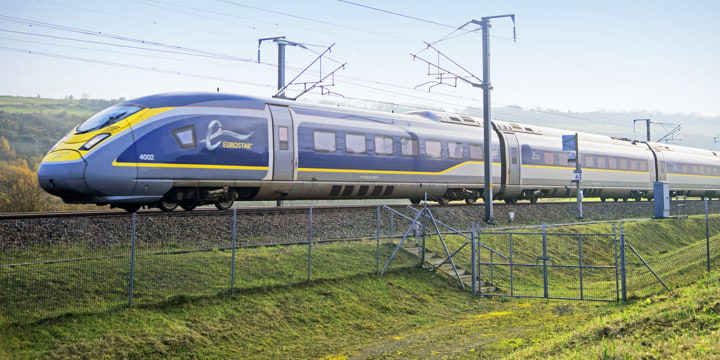This photograph captures a modern, high-speed Eurostar train viewed from a side angle, prominently featuring its aerodynamic, bullet-shaped design. The train’s front is adorned with yellow and blue hues, with "Eurostar" emblazoned in yellow letters, and an E-like design on the nose. The rest of the train exhibits a sleek mix of blue and gray, with visible windows and doors. The scene includes various elements: overhead wires and poles, a metal fence running along a grassy hillside, concrete steps, and a light blue sky forming the backdrop. Additionally, there is a gate-like structure situated down the hill on the right-hand side, adding depth to the setting.